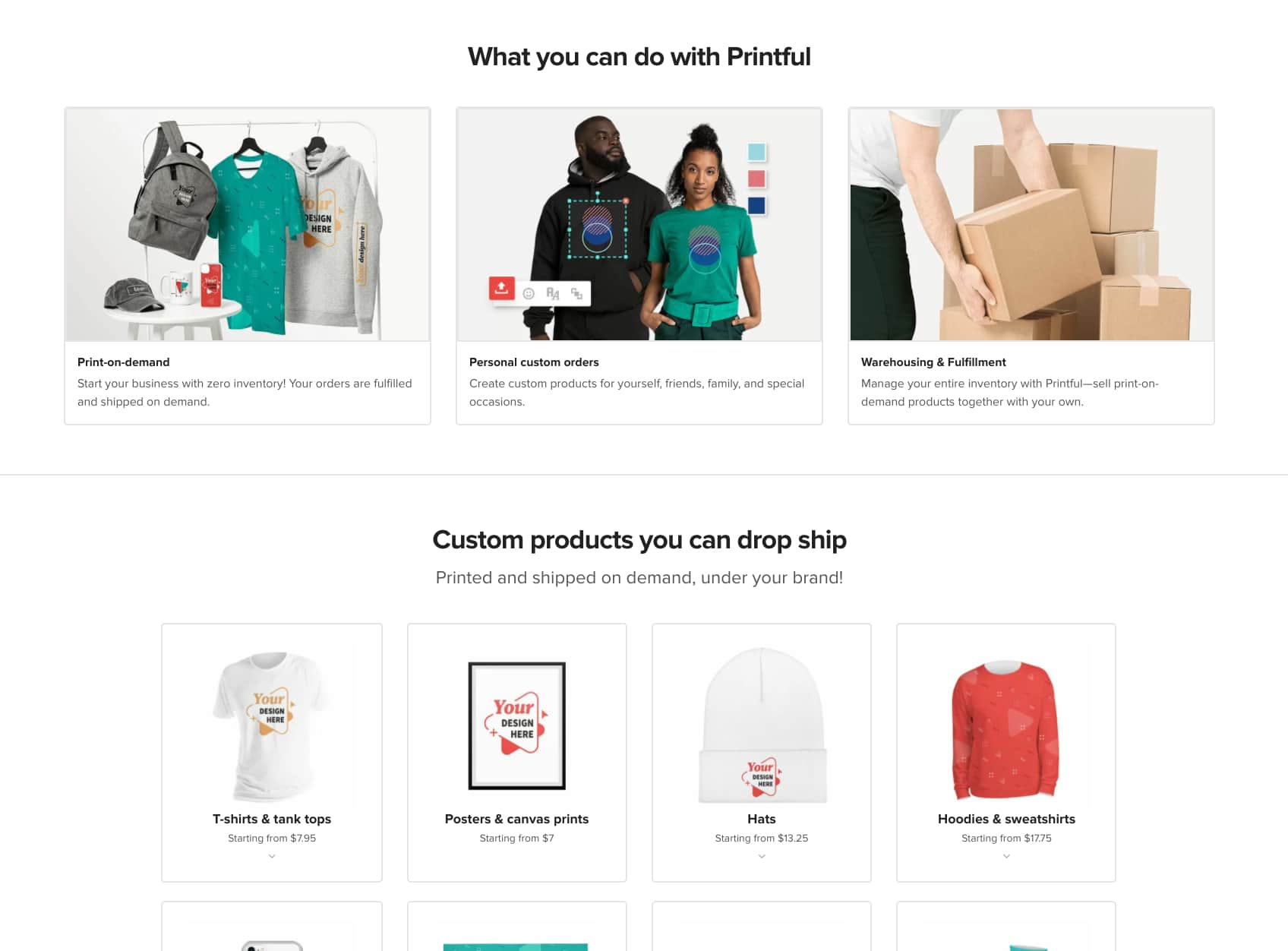The image captures a screenshot of a website that appears to be a platform for print-on-demand services, similar to Redbubble. The background is white, providing a clean and minimalist aesthetic. 

At the top of the website, there are three distinct square sections:

1. **Left Section:** This section emphasizes "Print on Demand," encouraging users to start their business with zero inventory. It highlights that orders are fulfilled and shipped on demand, indicating the website's focus on drop shipping.

2. **Center Section:** Here, the focus is on "Personal Custom Orders," where users are prompted to create custom products for themselves, friends, family, and special occasions. This section promotes the website’s ability to cater to personalized product needs.

3. **Right Section:** This section discusses "Warehousing and Fulfillment." It mentions that users can manage their entire inventory with the platform, specifically mentioning "Printful." The section points out that users can combine print-on-demand products with their own items.

Further down, another section directs attention to custom products available for drop shipping under the user's brand. The following information is provided for various products along with starting prices:
- T-shirts and tank tops starting at $7.95
- Posters and canvas prints starting at $7.00
- Hats starting at $13.25
- Hoodies and sweatshirts starting at $17.75

At the very bottom, the image is slightly cropped, revealing only four more tiles that are partially cut off, suggesting there are additional options or information beyond what is displayed.

This detailed breakdown showcases how the website aims to assist users in creating and managing custom products through print-on-demand and warehousing solutions.